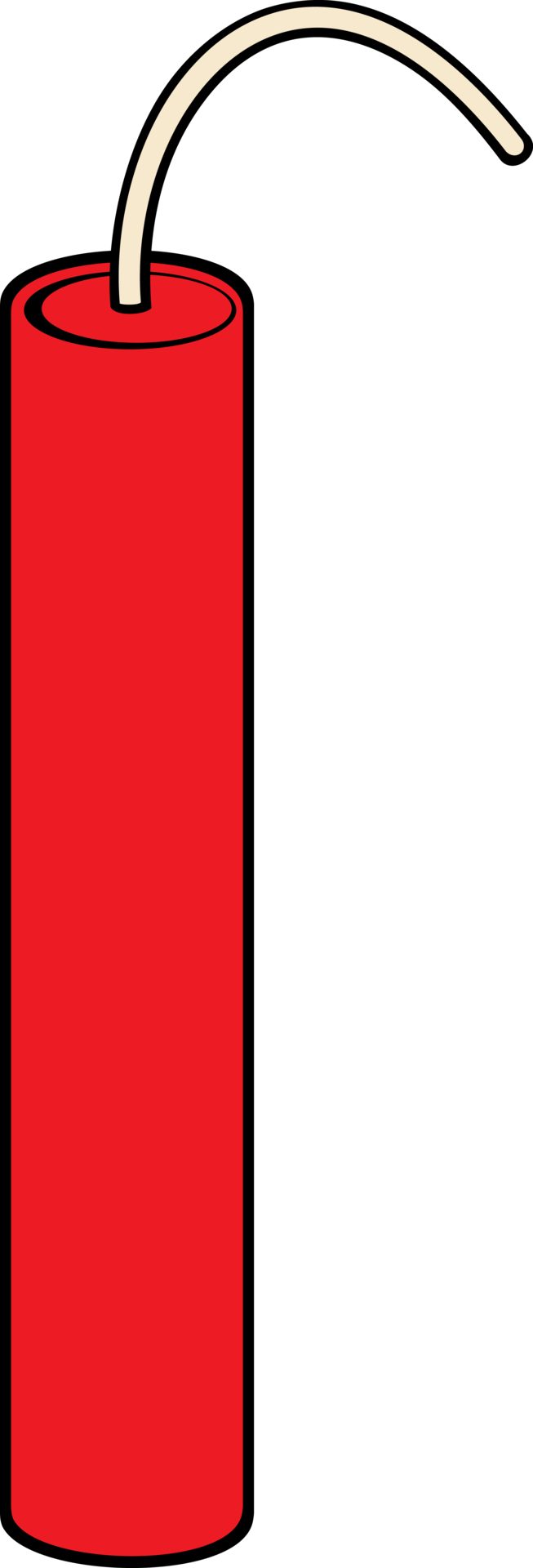The image is a vertically rectangular, simplistic print featuring a single stick of dynamite against a plain white background. The dynamite is rendered in a bold red color with a heavy black outline that traces the entire cylindrical body as well as the rounded top section. Emerging from the center of the top portion is a white fuse that curves slightly to the right, encased within the same black outline. The fuse is unlit and extends in a straw-like color. There are no additional markings, labels, or text on the dynamite, emphasizing its iconographic nature. The minimalist style highlights the clear shape and color contrast of the dynamite, making it unmistakably identifiable despite the lack of specific detail or labeling.